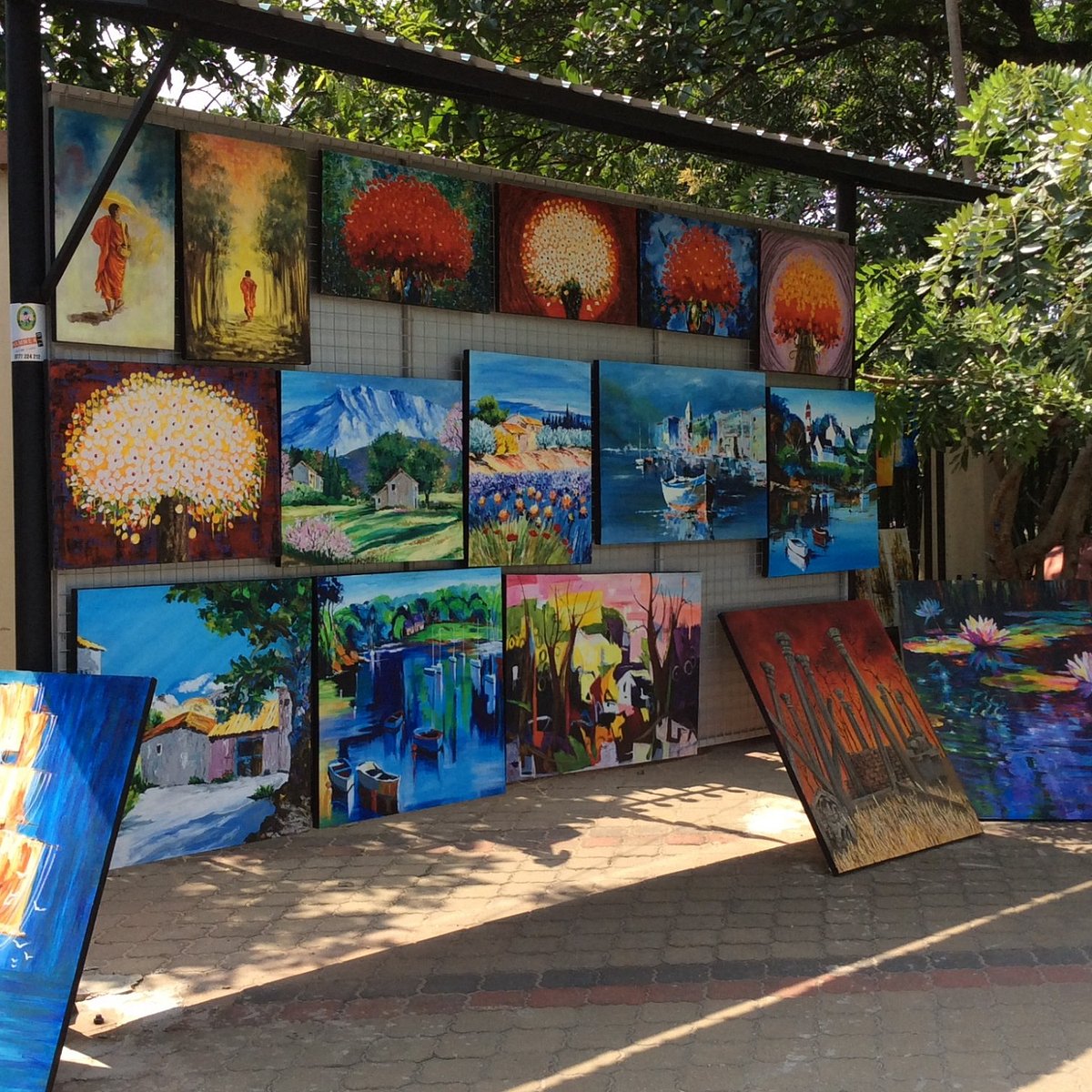The photograph captures a vibrant outdoor display of numerous acrylic paintings, amounting to about 14 or 16, arranged under a trellis on a pavement walkway, suggesting a street vendor or art festival setting. These colorful pieces, rich in reds, oranges, and blues, are mounted on a single panel with some paintings hung up in three rows, while several others lean against or are propped up on the ground. The art varies in style from surrealism to abstract, depicting a range of subjects including abstract trees, landscapes, mountain scenes with houses, seaports with boats, flowers, and people strolling in forests. A few standout pieces portray lily pads on a pond and diverse neighborhoods, all rendered with a dynamic, pop-art flair. In the background, the faint presence of trees adds to the outdoor atmosphere.